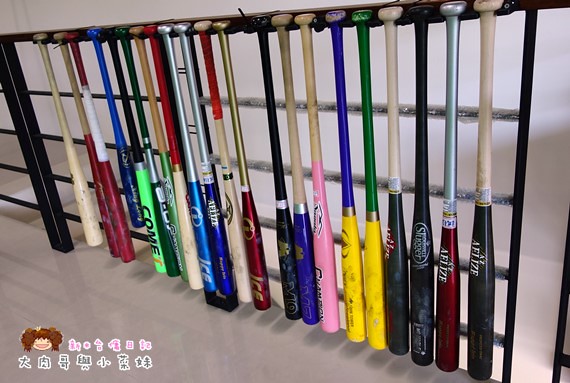This is an angled, color photograph taken indoors, depicting a tall, black metal rack holding 21 baseball bats of various colors. The bats, which include shades of yellow, pink, blue, green, red, purple, tan, and natural wood, are hung upside down by their handles on small black hooks at the top of the rack. The dual-colored design of many bats features different hues on the handle and the broader hitting end. The rack is freestanding against a pristine white wall and rests on a shiny, reflective white floor that mirrors the bats and the rack. In the bottom left corner of the image, there's a cartoon face of a smiling girl with curly brown hair, accompanied by Chinese characters.